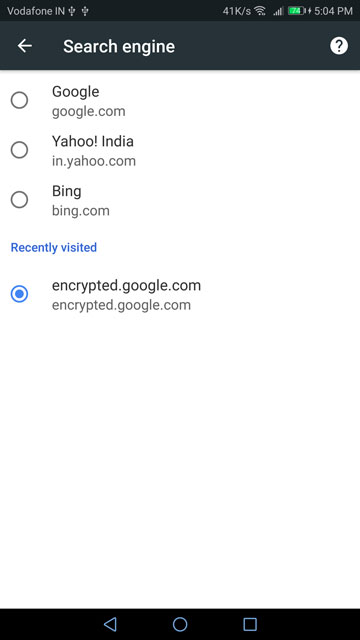A detailed screenshot is captured displaying a smartphone interface on a white background, with the notification bar indicating "IN" as the location and "5:04 PM" as the current time. A battery icon with a charge symbol is visible. Below this, there is a prominent gray rectangle containing a search engine selection screen.

The search engine selection interface features three options accompanied by radio buttons: "Google" with its URL google.com, "Yahoo" with its URL in.yahoo.com, and "Bing" with its URL bing.com. None of these options are currently selected. Additionally, there is a "Recently Visited" section which highlights another radio button that is checked in blue, corresponding to the URL encrypted.google.com, representing Google's encrypted search.

A black navigation bar is situated at the bottom of the screen containing three blue icons: a left-facing arrow shaped like a triangle, a circle, and a square, likely representing the back, home, and recent apps buttons respectively. A white circle with a gray question mark and three unselected radio dial buttons are also subtly displayed within the interface. The overall composition conveys the settings for selecting a preferred search engine on the device.